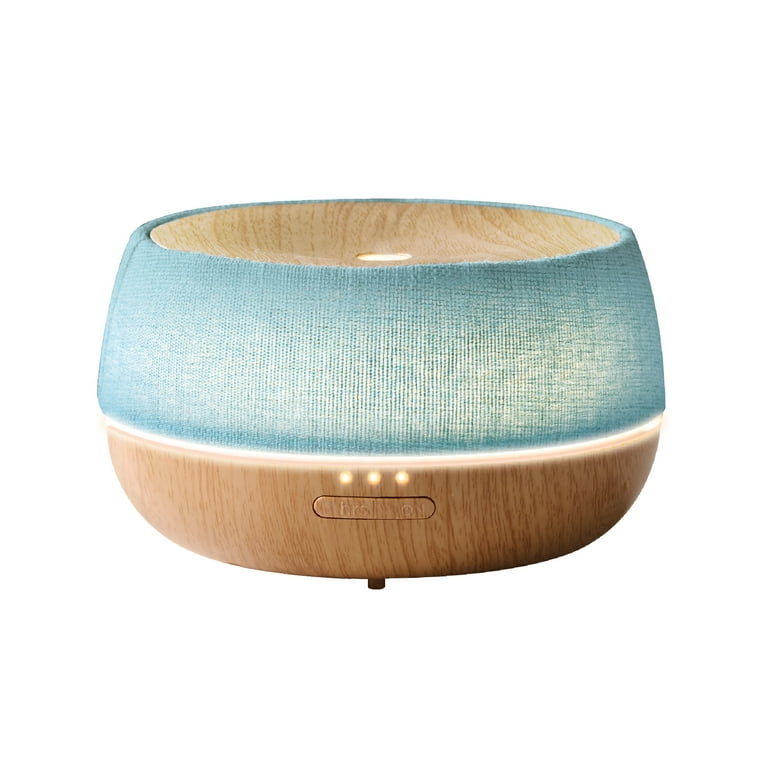This image showcases an object on a plain white background, appearing to be an oil diffuser or aromatherapy mister. The device is approximately four inches wide and about two inches high, with an additional half inch added by its rounded basin top. The depressed area of the top basin is finished in a light brown wood tone, featuring a center oval shape that appears round due to the angle.

The upper part of the diffuser is adorned with a light blue fabric, illuminated from the inside, giving it a semi-transparent appearance. A white light band runs horizontally across the center, accompanied by three small white illuminated dots underneath. The base of the diffuser retains the light brown wood tone, housing an oval button with raised print, inscribed with "HRS" on the left and "ON" on the right. A small, square foot is visible at the bottom of the diffuser, providing support.